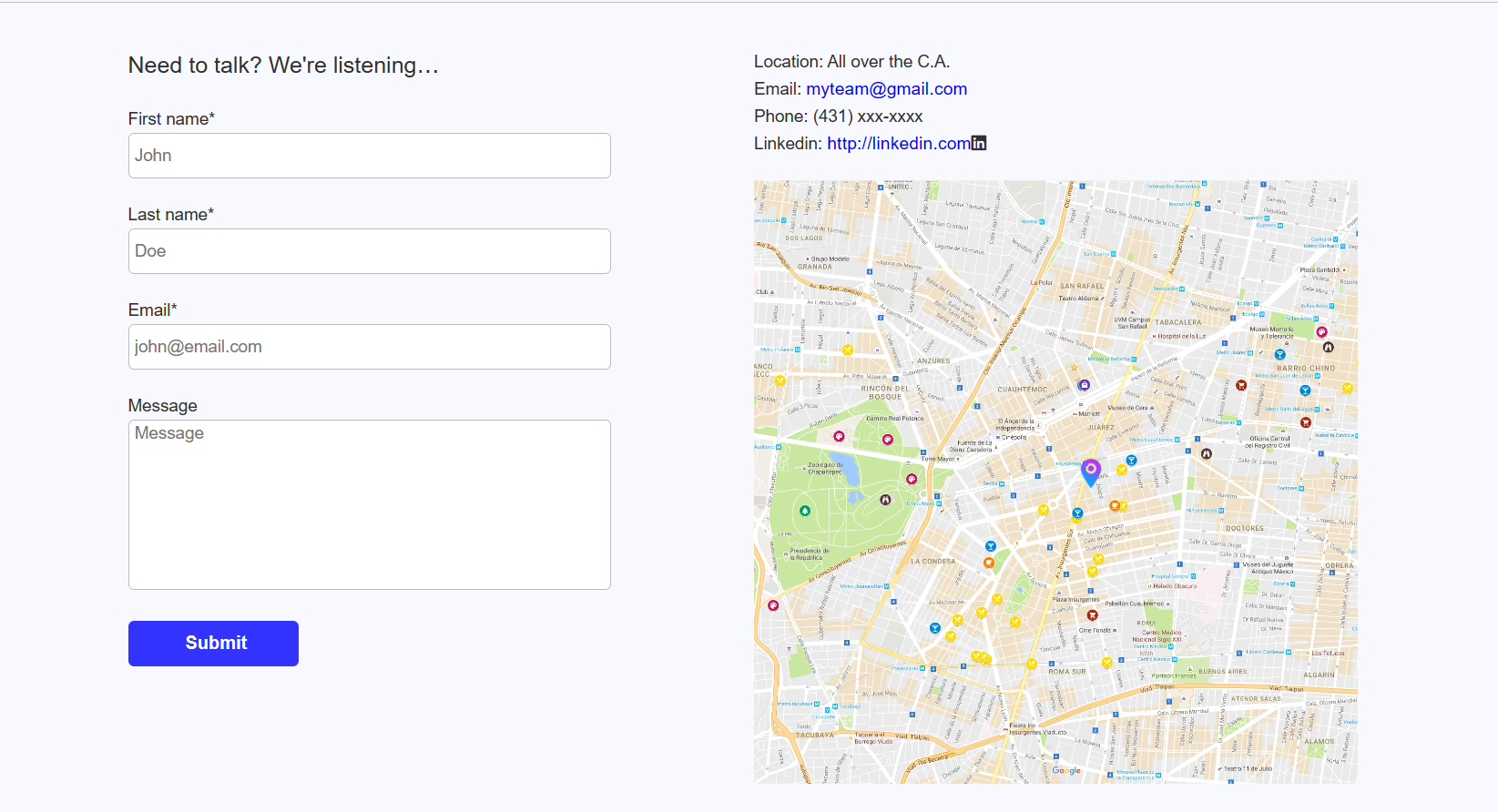The image features a slightly wider-than-usual square with a gray background. On the top left corner, the text in black reads, "Need to talk? We're listening...". Below this prompt, there is a form requesting user information with fields labeled "First Name," "Last Name," "Email" (each accompanied by an asterisk indicating required information), and "Message." Each field is represented by a white, blank space for the user to enter their details. 

At the bottom of the form, there is a prominent blue "Submit" button with the text "Submit" in white.

On the right side of the image, the following contact details are listed at the top: 
- "Location: All over CA"
- "Email: myteam@gmail.com"
- "Phone: (431) XXX-XXXX"
- "LinkedIn: http://linkedin.com"

Beneath this text, there is a map highlighting streets and landmarks in the area.